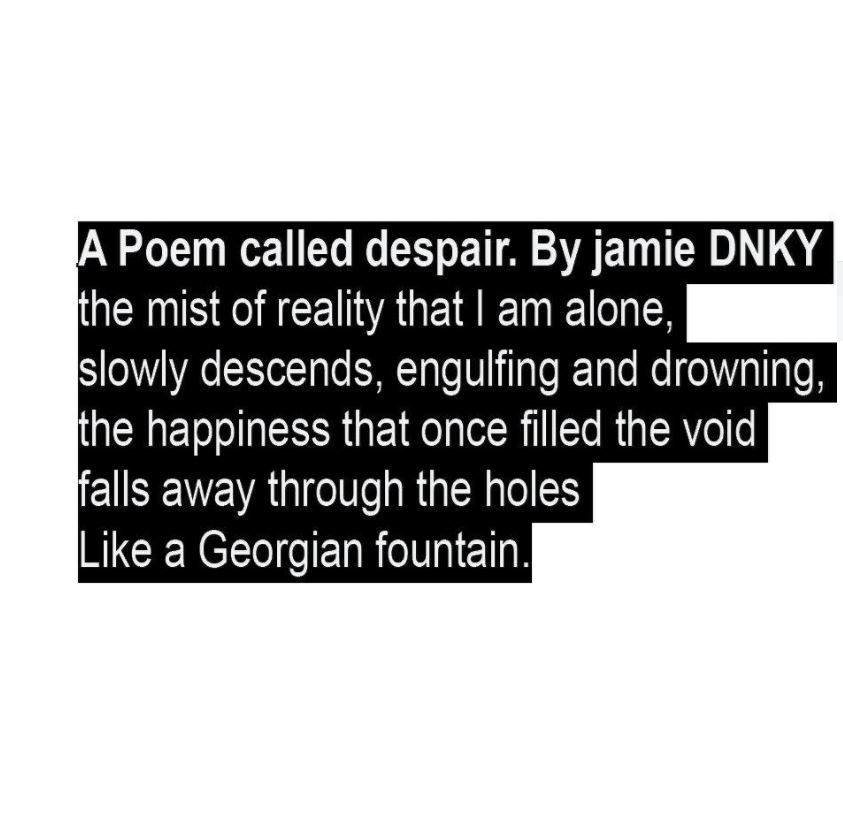This text image on a white background features a black rectangular box that highlights each of the six lines of white text, giving it the appearance of a meme. Titled "A Poem Called Despair" by Jamie DNKY, the title is formatted with 'Jamie' in lowercase and 'DNKY' in uppercase letters. The poem reads: "The mist of reality that I am alone slowly descends, engulfing and drowning the happiness that once filled the void. Falls away through the holes like a Georgian fountain." The overall tone of the poem is pessimistic, emphasizing feelings of isolation and the gradual loss of happiness.